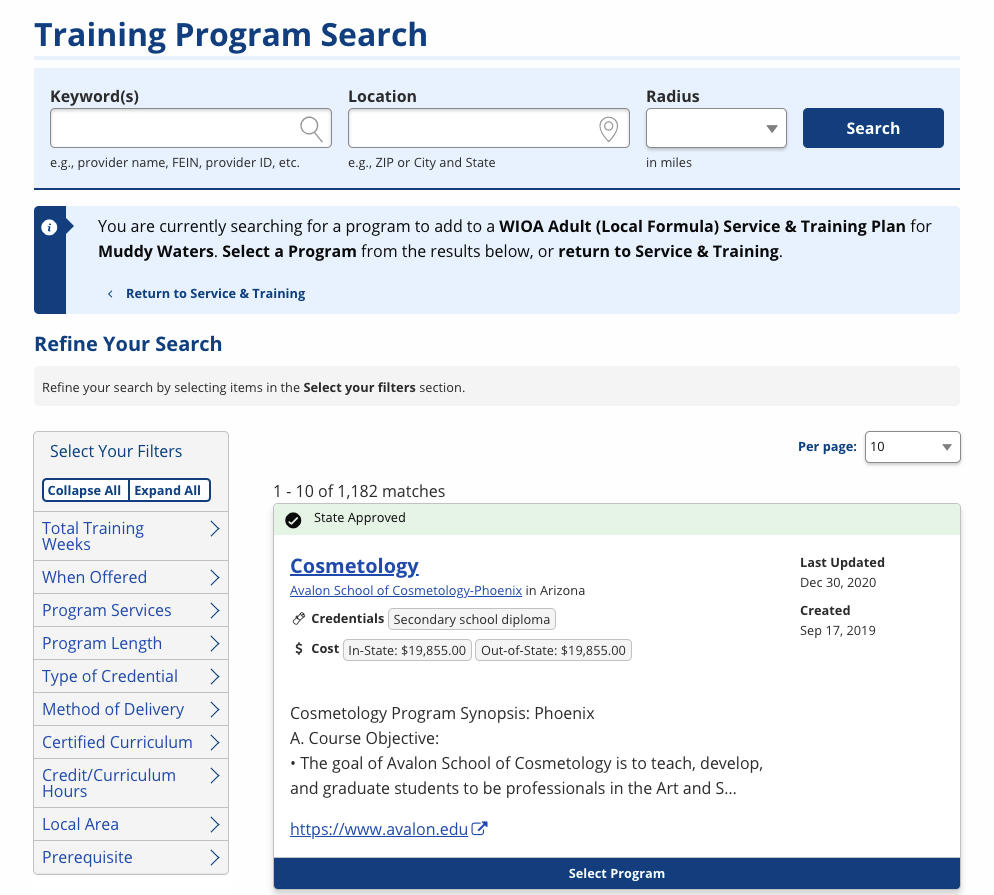In this image, we see a screenshot of a training program search interface. In the upper left-hand corner, the title "Training Program Search" is prominently displayed. Below that, there is a text box labeled "Keywords," with an example prompt suggesting inputs like "provider name, FEIN, provider ID, or UTC." The subsequent text box is labeled "Location" and includes example inputs such as "zip or city and state." Adjacent to the location box, there is a dropdown menu labeled "Radius in miles," allowing users to specify the search radius. Over to the far right, a distinctive blue "Search" button is positioned.

Directly beneath these search fields, a notification states, "You are currently searching for a program to add to a WIOA Adult Local Formula Service and Training Plan for Muddy Waters. Select a program from the results below. Return to service and training." Following this, there is an option to "Refine your search," guiding users to narrow their search by selecting items within the "Select your filter" section.

On the left side under "Select your filters," various filtering options are listed, which include: Total Training Weeks, When Offered, Program Services, Program Length, Type of Credential, Method of Delivery, Certified Curriculum, Credit Curriculum Hours, Local Area, and Prerequisite. On the right side of the interface, the results display a state-approved program titled "Cosmetology," offering courses at Avalon School of Cosmetology, located in Phoenix, Arizona.